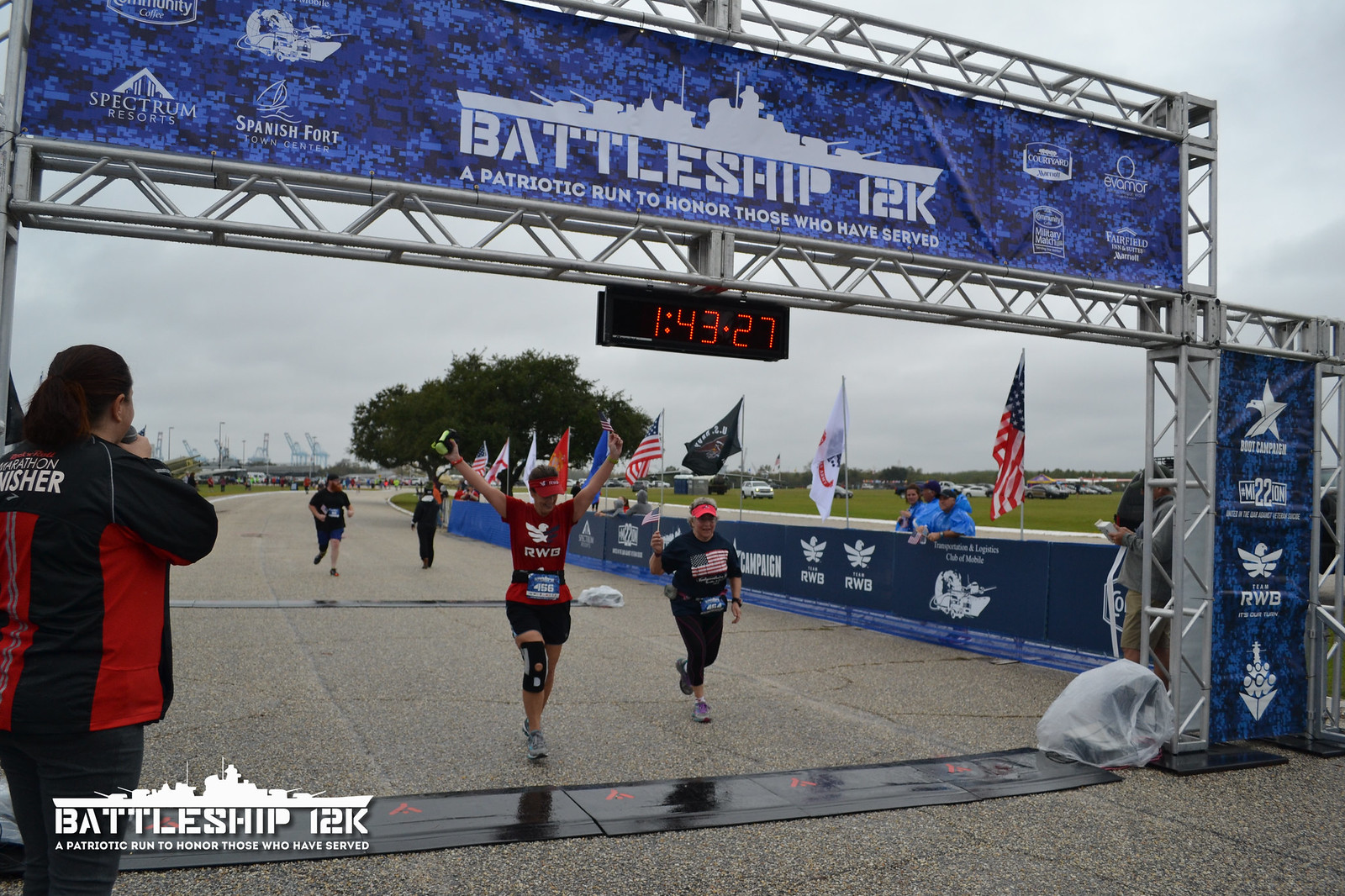The image captures the scene at the finish line of the Battleship 12K, a patriotic run to honor those who have served. The finish line is framed by steel girder beams, forming an opening with a banner overhead. The banner prominently displays "Battleship 12K" along with the phrase "A Patriotic Run to Honor Those Who Have Served." An outline of a battleship is positioned above the text. Timers showing a duration of 1 hour, 43 minutes, and 27 seconds are visible in red LED lights above the runners.

Two older women, about to cross the finish line, are at the forefront. One wears a red short-sleeved T-shirt, black shorts, a red visor, and a knee support, with her arms raised triumphantly. The other woman dons a black T-shirt featuring an American flag, black leggings, trainers, and a red visor, holding a small American flag in her hand. Behind them, a man with a beard and glasses wears a black cap and is steadily making his way to the finish line.

The stands hold a few spectators, some of whom are seated under flags. On the far side of the finish line, an official is present holding a microphone, presumably to announce the finishers. Sponsors' logos are visible on both sides of the finish line structure, contributing to the event's patriotic atmosphere.